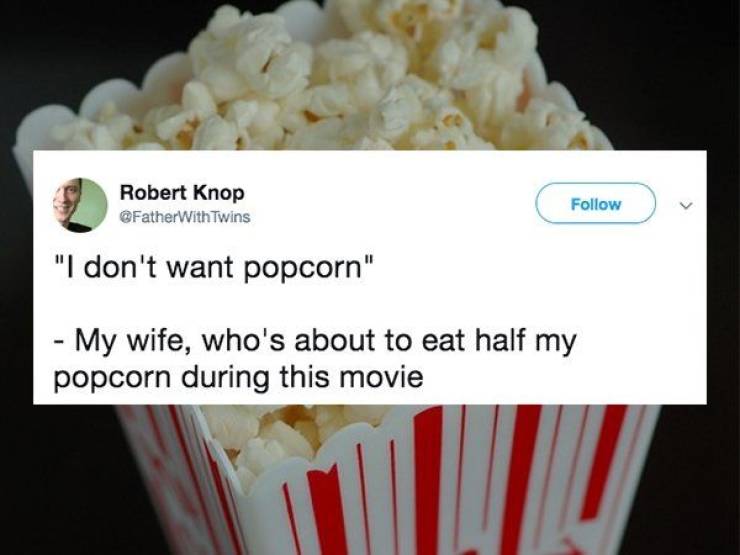In this image, a traditional red and white striped popcorn container overflowing with light yellow popcorn is prominently displayed against a black background. The focal point of the image is a social media screenshot overlaying the popcorn, shared by Robert Knopp, which humorously reads: "I don't want popcorn, my wife, who's about to eat half my popcorn during this movie". The screenshot, resembling a Twitter post with a blue "follow" button and a small green profile picture showing part of a man's face, adds a humorous contrast to the image. The colors in the composition include red, white, light yellow, black, blue, and green, creating a visually engaging and comedic scene that evokes the experience of sharing popcorn at a comedy movie. Everything is well-centered, with the tweet positioned right in the middle, making the overlay the central element drawing the viewer's attention.